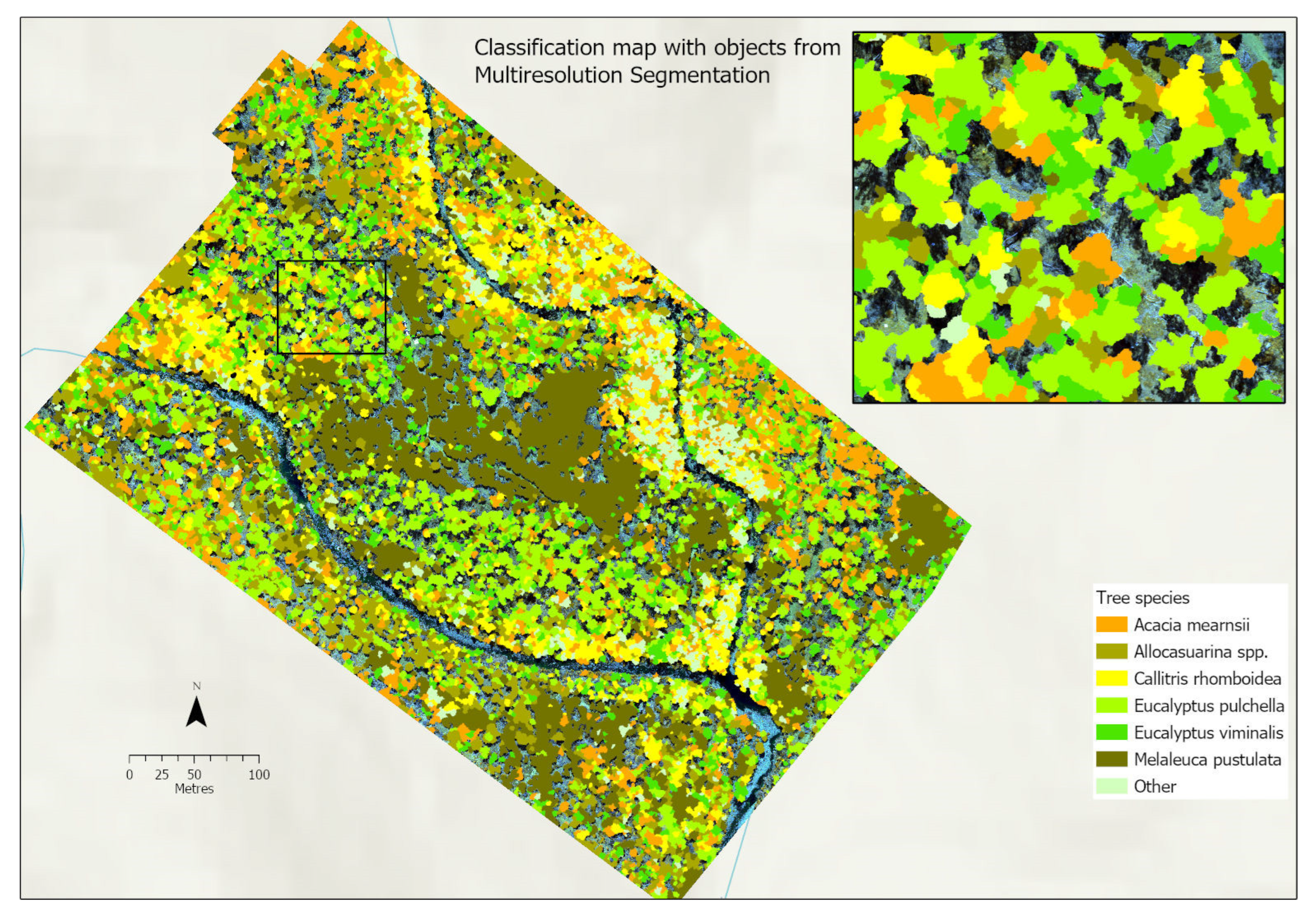The image is a detailed classification map with objects from multi-resolution segmentation, highlighting various tree species in a specific area. The map is divided by a river into three sections and uses a variety of colors to denote different tree species. The colors include neons, greens, oranges, yellows, blues, blacks, grays, and beiges. The top left section of the map shows a diagonally placed rectangular image dotted with blobby shapes in these colors, while the top right features a close-up version displaying the same color-coded segmentation. The bottom section includes a key within a white square, specifying that orange represents Acacia myrnsi, olive green indicates Alocasurina spp, yellow denotes Kellytris rhomboidea, light green stands for Eucalyptus pulchella, regular green for Eucalyptus viminalis, dark olive green for Melaleuca pistulata, and light blue for other species. There's also a scale measuring distances and detailed labels indicating tree species names.